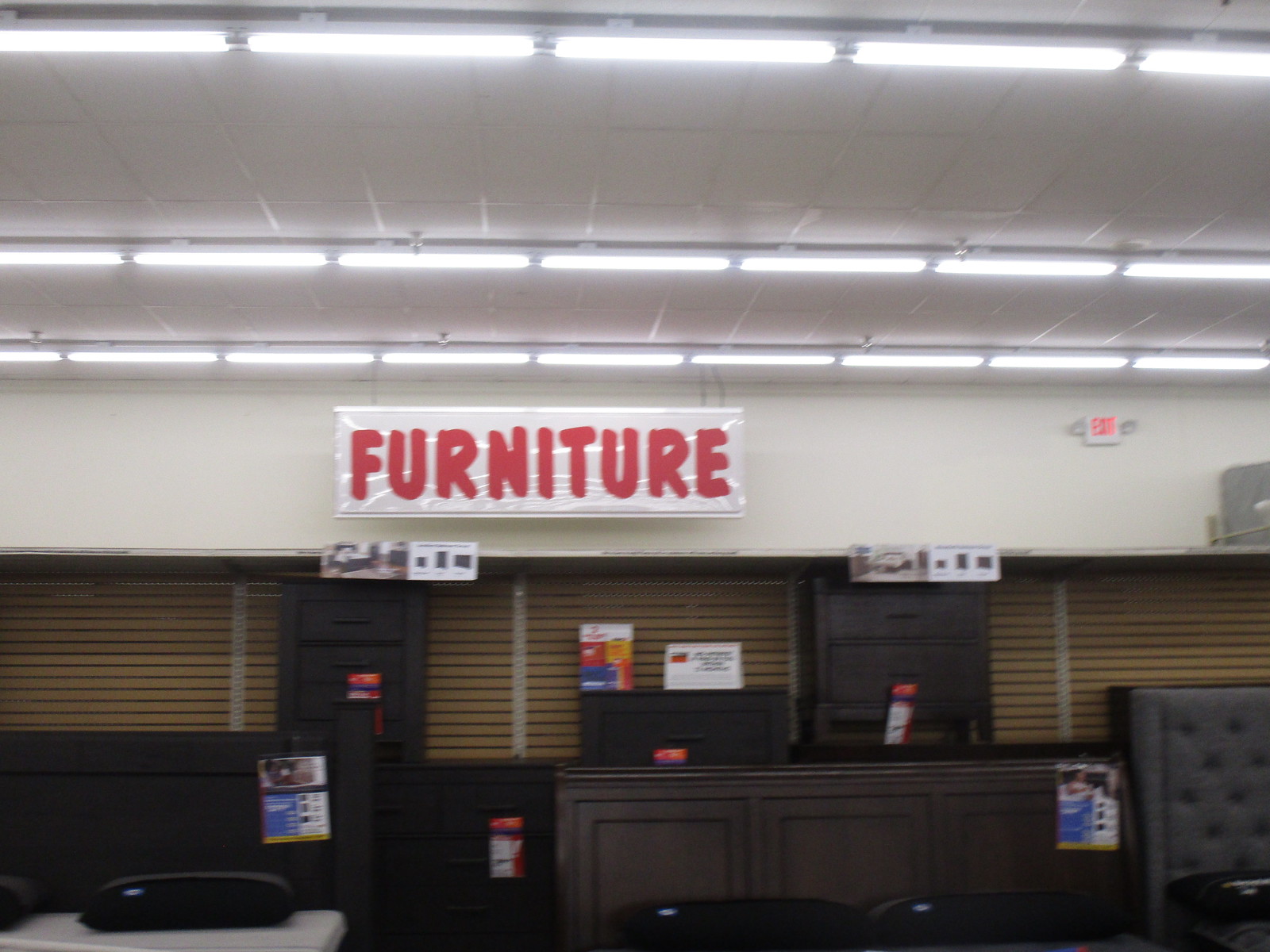The digital photo depicts the front interior section of a furniture store. The store features a white drop ceiling with bright fluorescent lights running horizontally across the top part of the image. Prominently displayed in the center, hanging from the ceiling, is a large white banner-style sign with the word "FURNITURE" written in bold red capital letters with rounded edges. Below the sign, several pieces of furniture are arranged on the ground, including black dressers, nightstands, and a gray tufted bed frame. A mattress is visible at the bottom left, paired with a dark pillow. Additionally, there are wooden blinds covering the glass windows in the background, and each furniture piece has an information or pricing sheet. Towards the right side of the image, an emergency light and a red exit sign are visible on the white wall.